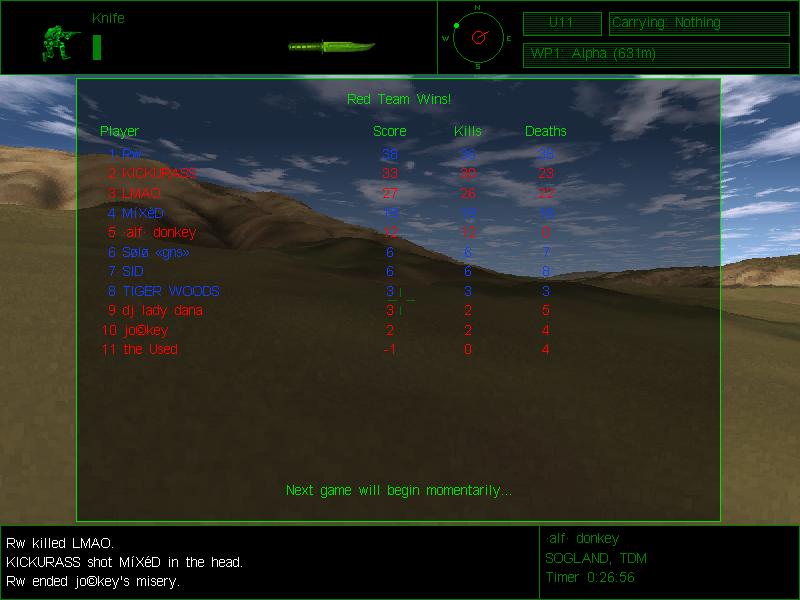This screenshot from a probable Steam PC game, possibly a first-person shooter played in teams, showcases a detailed interface against a desert landscape with a bright blue sky and wispy clouds. Central to the image is a translucent menu displaying, "Red Team Wins," highlighting the scores, kills, and deaths for 11 players. Their names, like Used, Jockey, and DJ LadyClaria, are shown in blue and red to signify their respective teams. At the bottom of this menu, it states, "Next game will begin momentarily." 

Overlaying the background is a navigation bar with a green outlined soldier icon labeled "knife" next to a small green bar. Below this is a green knife icon, a compass pointing slightly west, and additional information, "U-11, carry nothing, WPI alpha, 631 meters." A black box on the left reads, "ALF DUNKEY SOGLAND TDM timer 2656."

At the bottom, game commentary includes, "RW killed LMAO, Kick your ass shot mixed in the head, RW ended jockey's misery," indicating player actions. This elaborate setup not only shows the competitive nature of the game but also the intricate details used within the gaming interface.